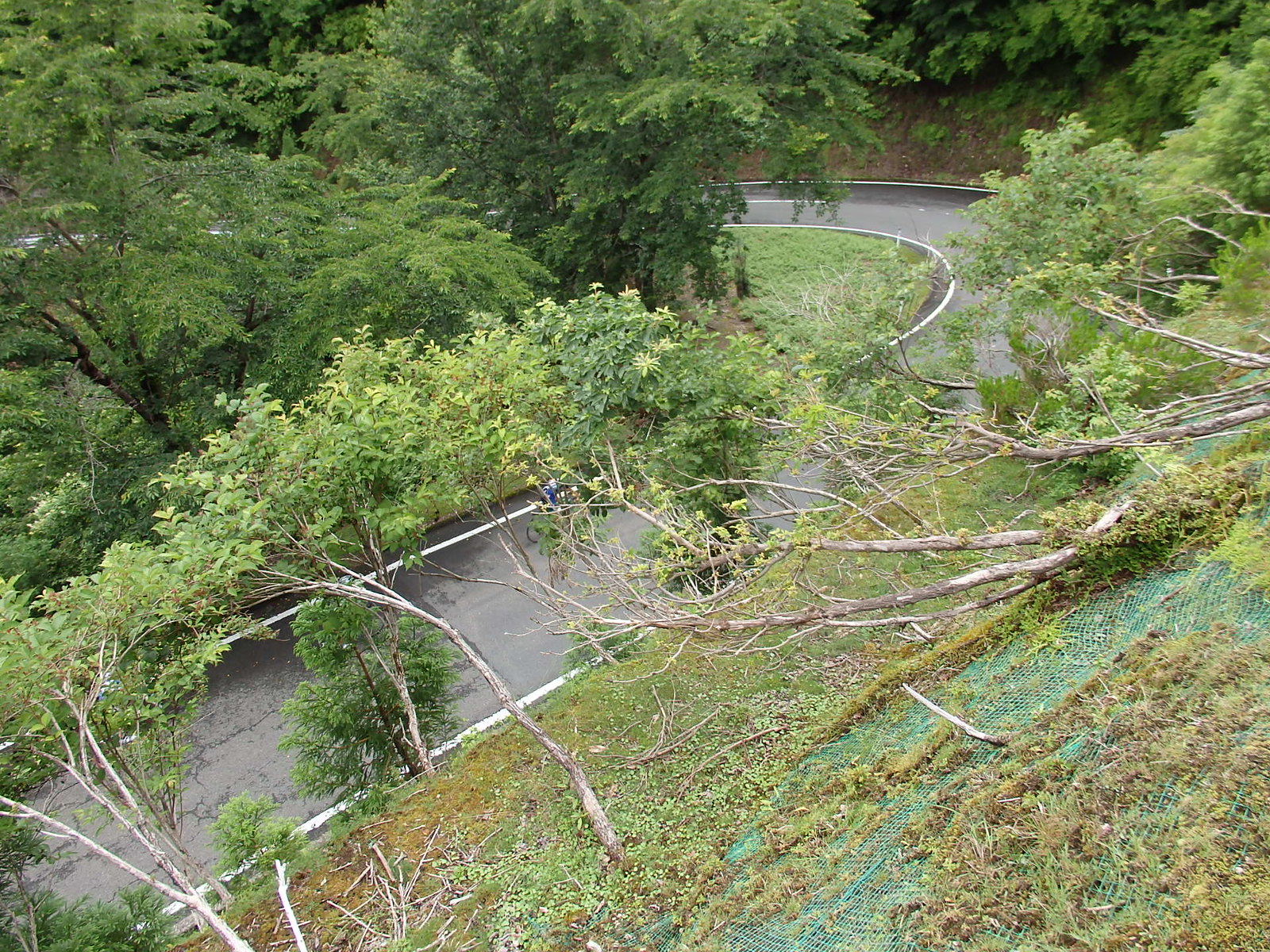This image is a detailed color photograph showcasing a winding, mountainous road from an overhead perspective. The road, which is gray and paved, features white lines outlining its edges, and it meanders through a lush landscape marked by abundant trees and vegetation. The winding path begins at the bottom left of the image, curving up towards the top right before bending back to the left, resembling a horseshoe curve. 

The road is devoid of vehicles but includes a single cyclist dressed in blue biking attire. The foreground reveals numerous tree branches with green and yellowish leaves, and the ground below shows a mix of gray, green, brown tones, and straw. The sides of the road display green netting, likely used for erosion control to prevent vegetation from sliding down onto the roadway.

Looking down from a higher vantage point, you can see not only the intricate curves of the road but also the tops of several trees indicating the varying elevation of the terrain. The upper part of the photograph showcases dense clusters of trees and foliage, underlining the road's mountainous setting.